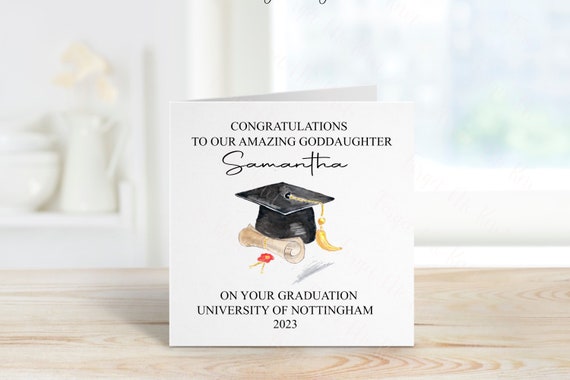In the center of the photograph, a white congratulatory card stands upright on a wooden surface. The card displays a heartfelt message in black text: "Congratulations to our amazing goddaughter, Samantha." Below this, in elegant cursive, her name, "Samantha," is highlighted. A prominent black graduation cap with a gold tassel is illustrated beneath her name. Accompanying this is a rolled-up certificate tied with a multicolored ribbon including red, pink, and yellow hues. At the bottom of the card, the inscription reads: "On your graduation, University of Nottingham, 2023."

The backdrop of the scene includes a plain white wall with a window to the right. On the left, there is a shelf holding a white picture frame and a vase filled with white flowers, next to a white bowl with a lid. These elements together create an elegant and celebratory atmosphere honoring Samantha’s achievement.